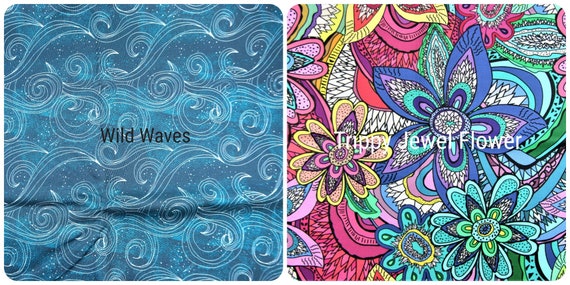The image features two square artworks with rounded corners, each showcasing distinct designs and color palettes. On the left, the piece titled "Wild Waves" displays an intricate pattern of swirling lines in white against a backdrop of dark and light blues, resembling turbulent ocean waves. The fabric has some wrinkles towards the bottom, adding texture to the overall composition. On the right, "Trippy Jewel Flower" is vibrant and retro, presenting an array of jewel-like flowers in colors including blues, yellows, pinks, and greens. The background is a mix of black and white, with many areas meticulously filled in with bold, lively hues.